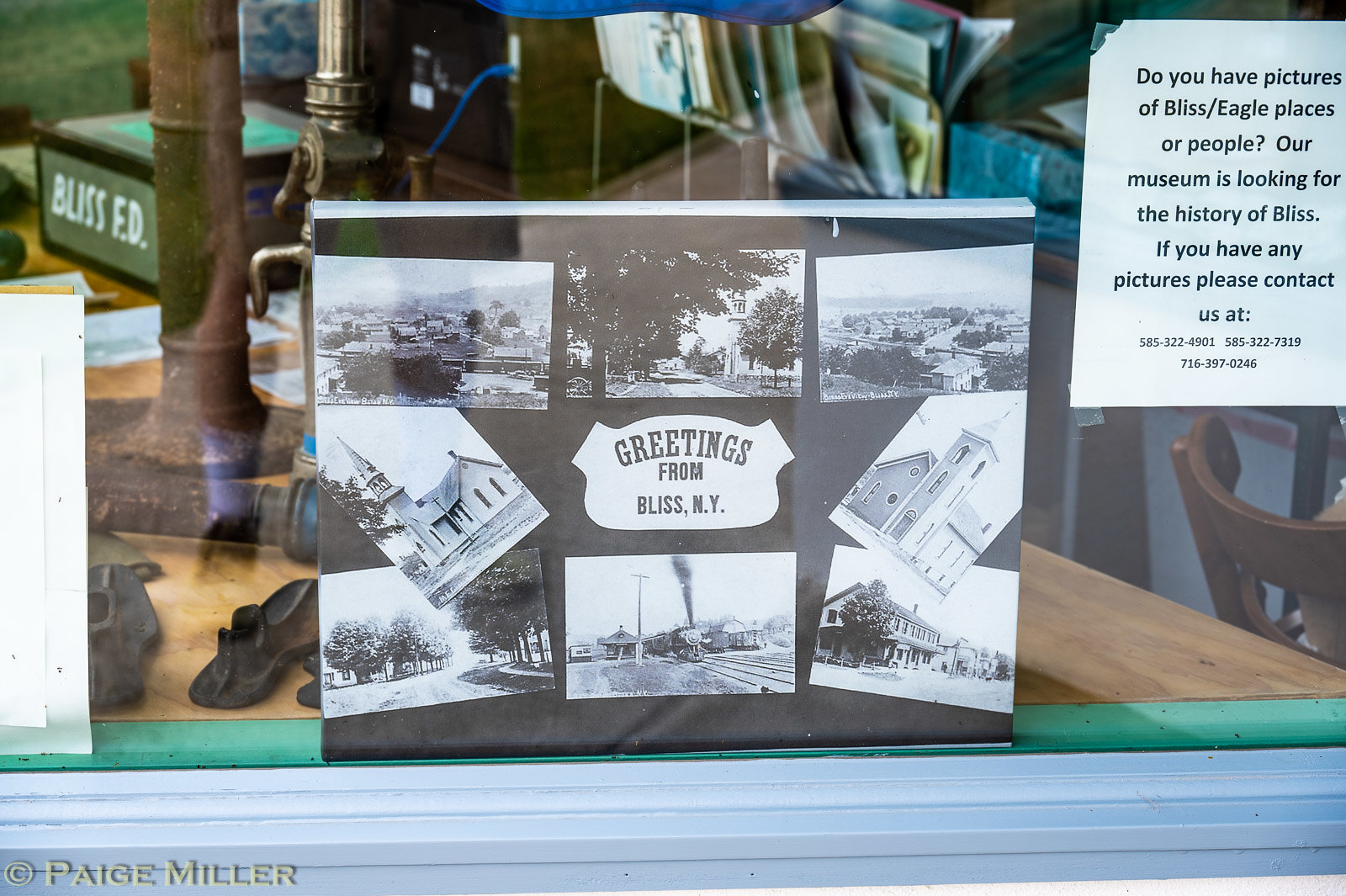In the center of the storefront window, a blackboard collage proudly displays black and white photographs of an old-time rural town, aptly labeled "Greetings from Bliss, NY" in bold black text. These images prominently feature a church and various vintage scenes from Bliss, New York. To the right of the collage, a piece of white paper with black printed text is taped to the window. The notice reads: "Do you have pictures of Bliss, Eagle Places, or People? Our museum is looking for the history of Bliss. If you have any pictures, please contact us at 585-322-4901, 555-322-7319, or 716-397-0246." The interior visible beyond the window reveals a long table adorned with antiques, including rusty metal items, an old phone, and some weathered shoes. The scene is framed by reflections on the windowpane, adding a layer of historical ambiance to the quaint display.